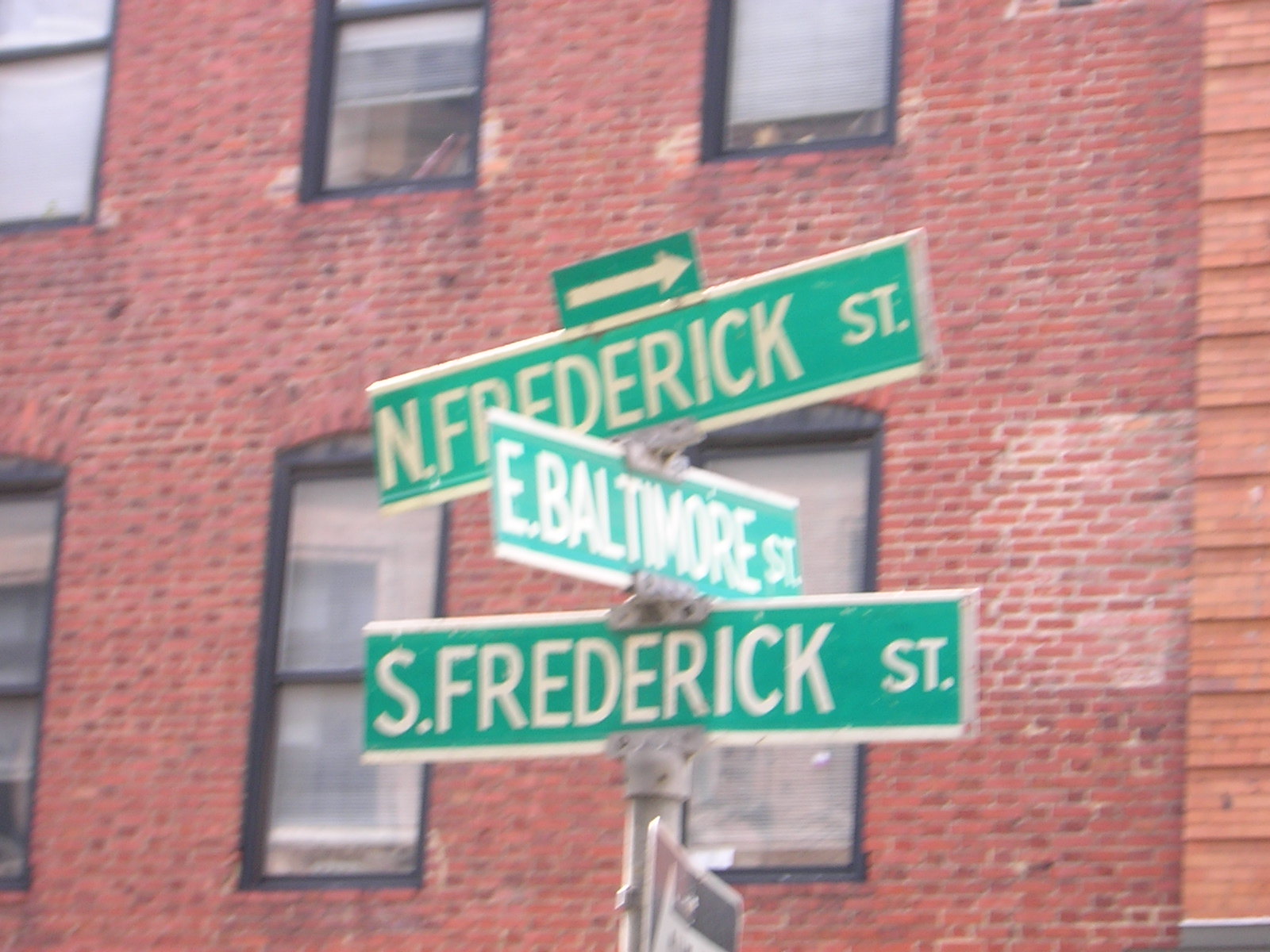This image captures a detailed view of an old, reddish brick building with a distinctive architectural style. The building is prominently featured, showing a variety of bricks, including a lighter shade forming a ladder-like pattern on the far right. It's at least two stories tall, with tall, black-framed sash windows that arch at the top and are situated close together. Some windows have partially open blinds, while others are fully open or closed.

In front of the building stands a metal post with three traditional green and white street signs arranged one above the other. At the top, a sign reads "North Frederick Street," with an arrow pointing to the right. Below it, another sign perpendicular to the others reads "East Baltimore Street," indicating the roadway. At the bottom, a sign says "South Frederick Street," implying a leftward direction. Beneath these, a barely visible one-way sign suggests East Baltimore Street is a one-way road.